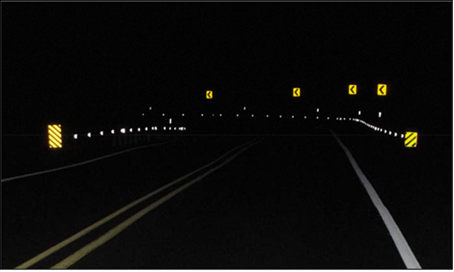This nighttime landscape photo captures a two-lane highway from the dashboard perspective of a vehicle. The road is mostly obscured in darkness, with visibility extending no more than ten feet ahead. The central double yellow lines and the single white lines on either side of the road are faintly illuminated. The road curves sharply to the left, as evidenced by reflective white markers lining the guardrails and multiple yellow signs with black arrows indicating the turn. Diagonal black-striped yellow rectangular signs further announce the curve. The photo's overall atmosphere is one of deep shadow, with the reflectors and signs providing the only guidance through the pitch-black surroundings.